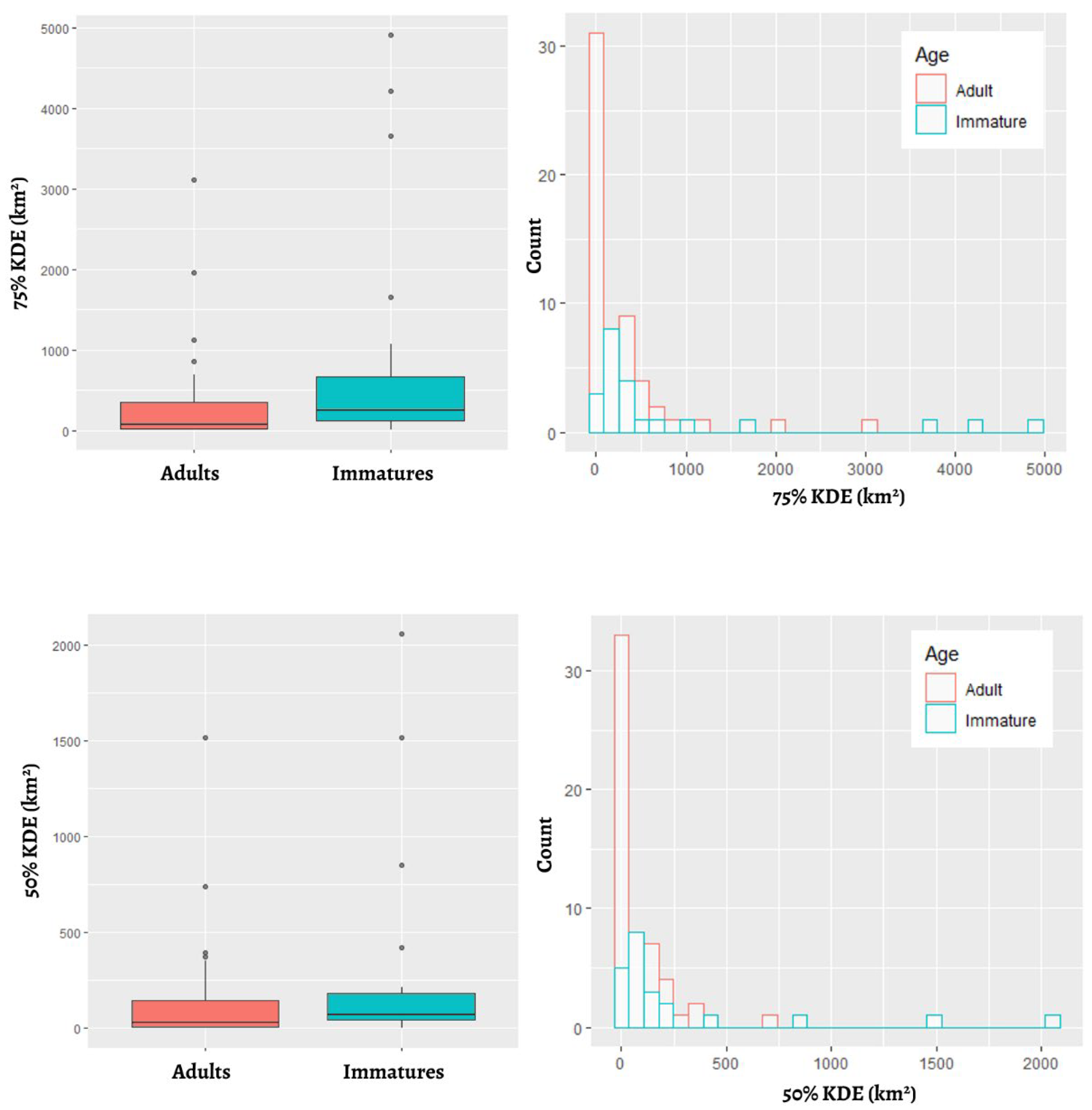The infographic is a color illustration comprised of four gray squares arranged in a 2x2 grid, used to convey detailed information about KDA (kilometers squared) distributions. The top left square is labeled "75% KDE KM2" and features a short orange bar for adults and a slightly larger turquoise bar for immatures, indicating that immatures have a higher count in this specific metric. The top right square serves as a legend with the title "Count" and labels for "75% KDE KM2," clarifying that adults are represented in red/orange and immatures in blue/turquoise. The bottom left square, labeled "50% KDE KM2," displays an almost equal comparison between adults and immatures with their respective bars, showing minimal difference in counts. The bottom right square, also labeled "Count, 50% KDE KM2," reinforces this comparison. Overall, the infographic highlights that adults have higher counts than immatures when totaling over 30 units, contrasting the two age groups in both 50% and 75% KDE metrics, depicted through individual and charted bar graphs.